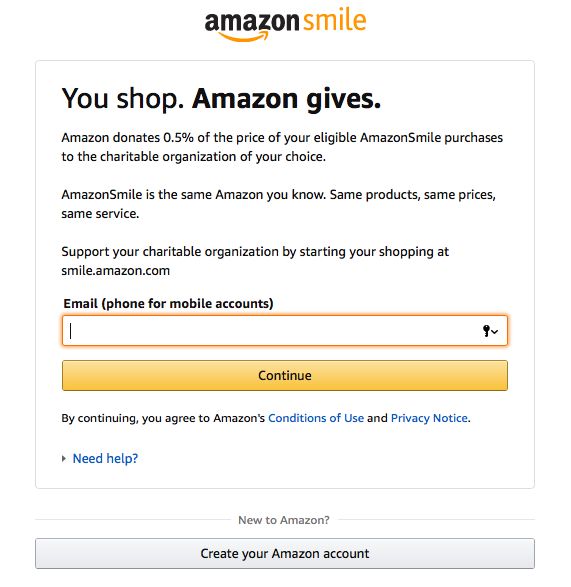Here is a cleaned-up and descriptive caption for the image:

"A detailed screenshot of the Amazon Smile program page. The top section features the iconic Amazon smile logo in orange with 'Amazon' in black text. Below, in a white box, the text reads: 'You shop. Amazon gives,' with 'Amazon gives' in bold. Following this is an explanatory paragraph in regular black text: 'Amazon donates 0.5% of the price of your eligible Amazon Smile